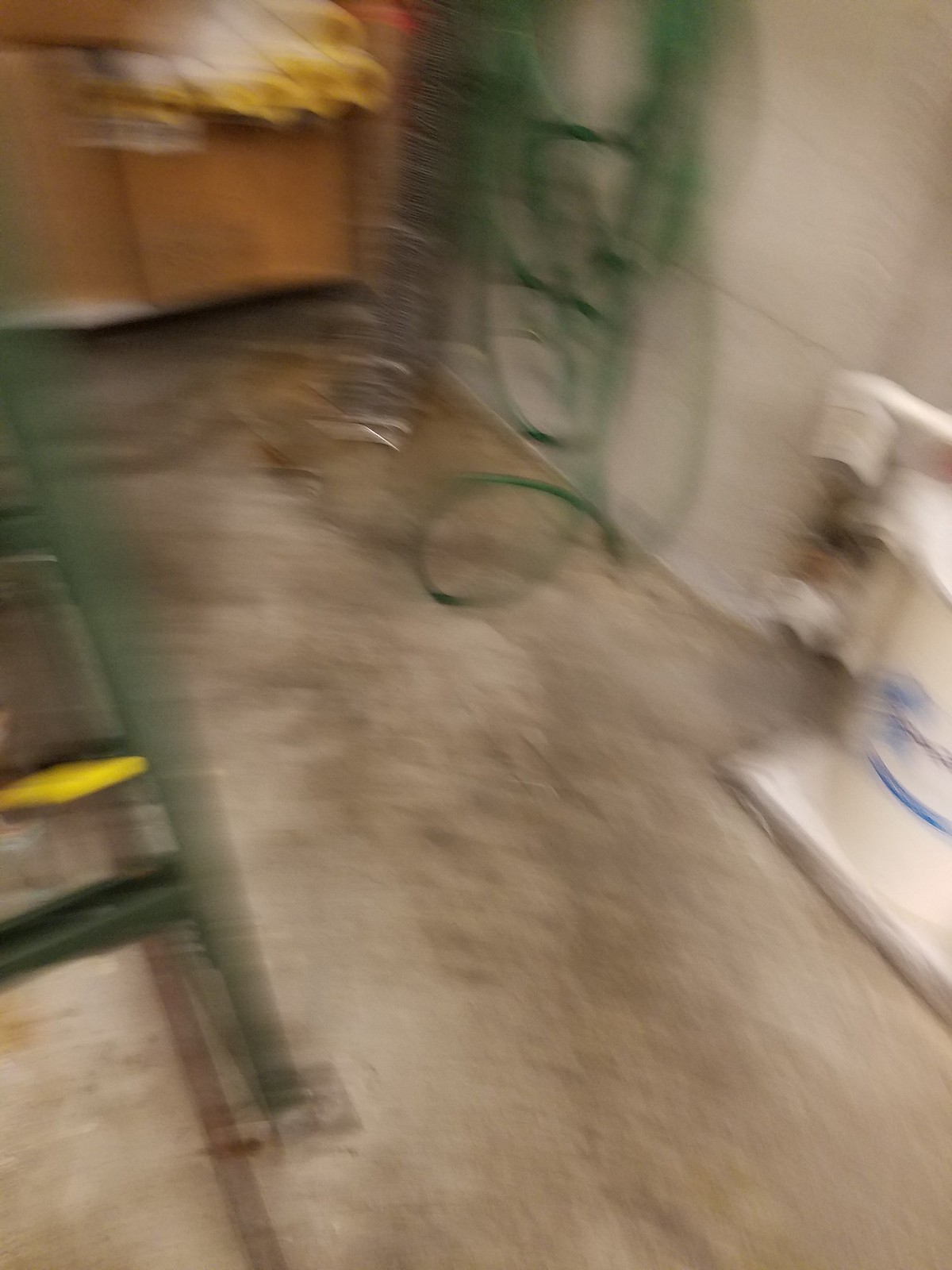The image is an extremely blurry photograph taken indoors, possibly in a garage, basement, or storage room. The scene includes a dirty concrete floor littered with stains and dirt. In the top background, there is a brown area resembling wooden shelves holding assorted objects. The right side is dominated by a white concrete or tile wall, with a green object hanging from it that appears to be a garden hose or wiring. In the bottom left corner, part of a green ladder with a yellow step is visible, and the bottom right features a white metal device with a blue line running down the middle. Additionally, there seem to be pipes and possibly bags near the white device, contributing to the sense of clutter and disorganization. Overall, the image suggests a functional but untidy storage or utility space.